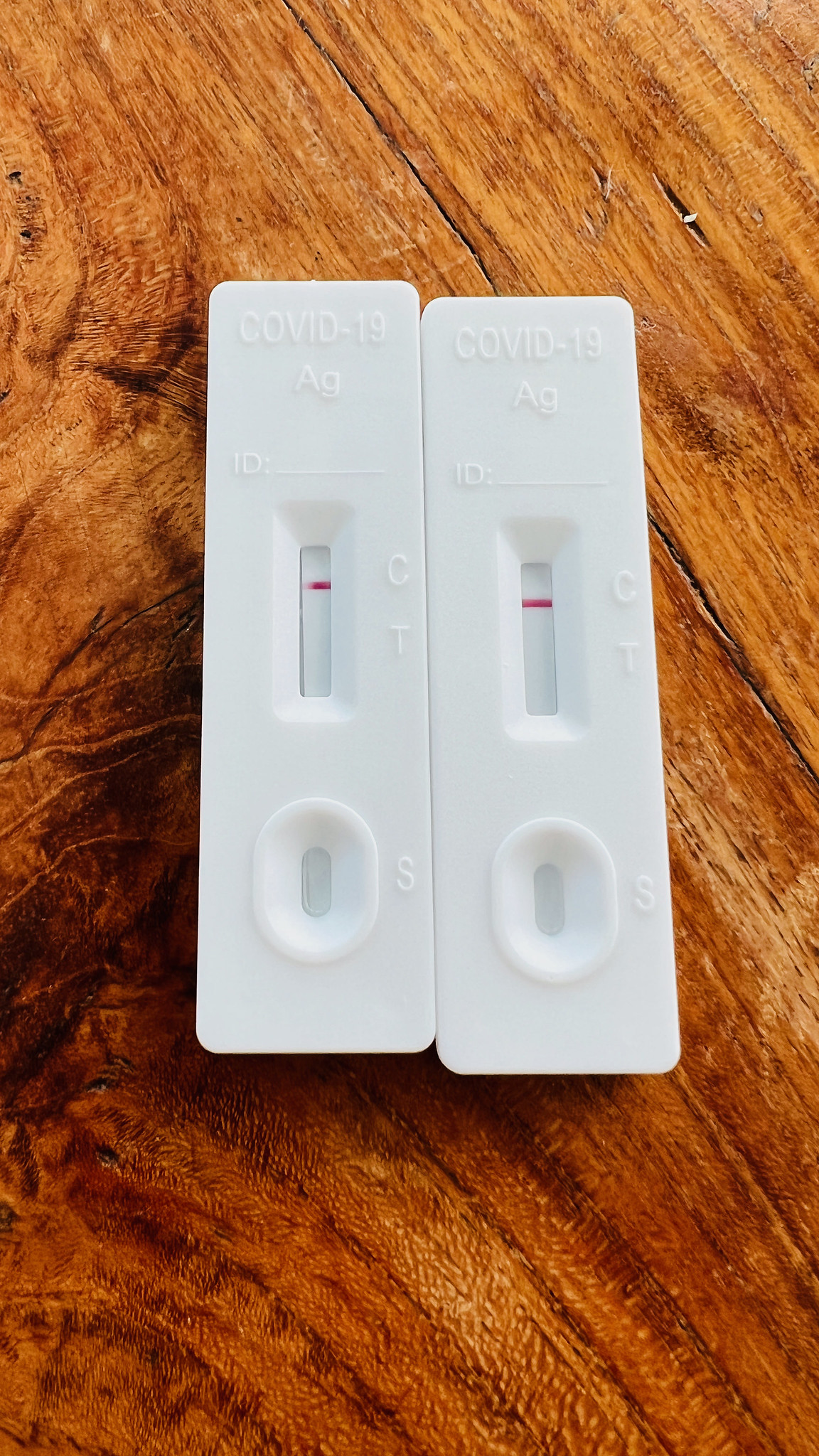The image depicts a vertically oriented, rustic brown rectangular table, exuding a farmhouse charm with its rich texture and intricate wood grains. The table showcases a variety of markings—nicks, notches, darker patches, and unique edges—that accentuate its authenticity and character. A subtle reddish tint adds depth to its rustic appearance. 

In the center of the table lie two white COVID-19 tests, positioned side by side but slightly misaligned, with the one on the right sitting marginally lower than the other. Both tests are labeled with raised, plasticky white letters reading "COVID-19" followed by "A-G" and "ID:". Each test features a small rectangular display area with marked "C" and "T" indicators. The presence of a pink line next to the "C" on both tests signifies a certain test result. Below the display area is an oval slot, encased in a thicker white border, labeled with an "S" on each test. The juxtaposition of the modern, clinical COVID-19 tests against the backdrop of the rustic table creates a striking contrast in the image.